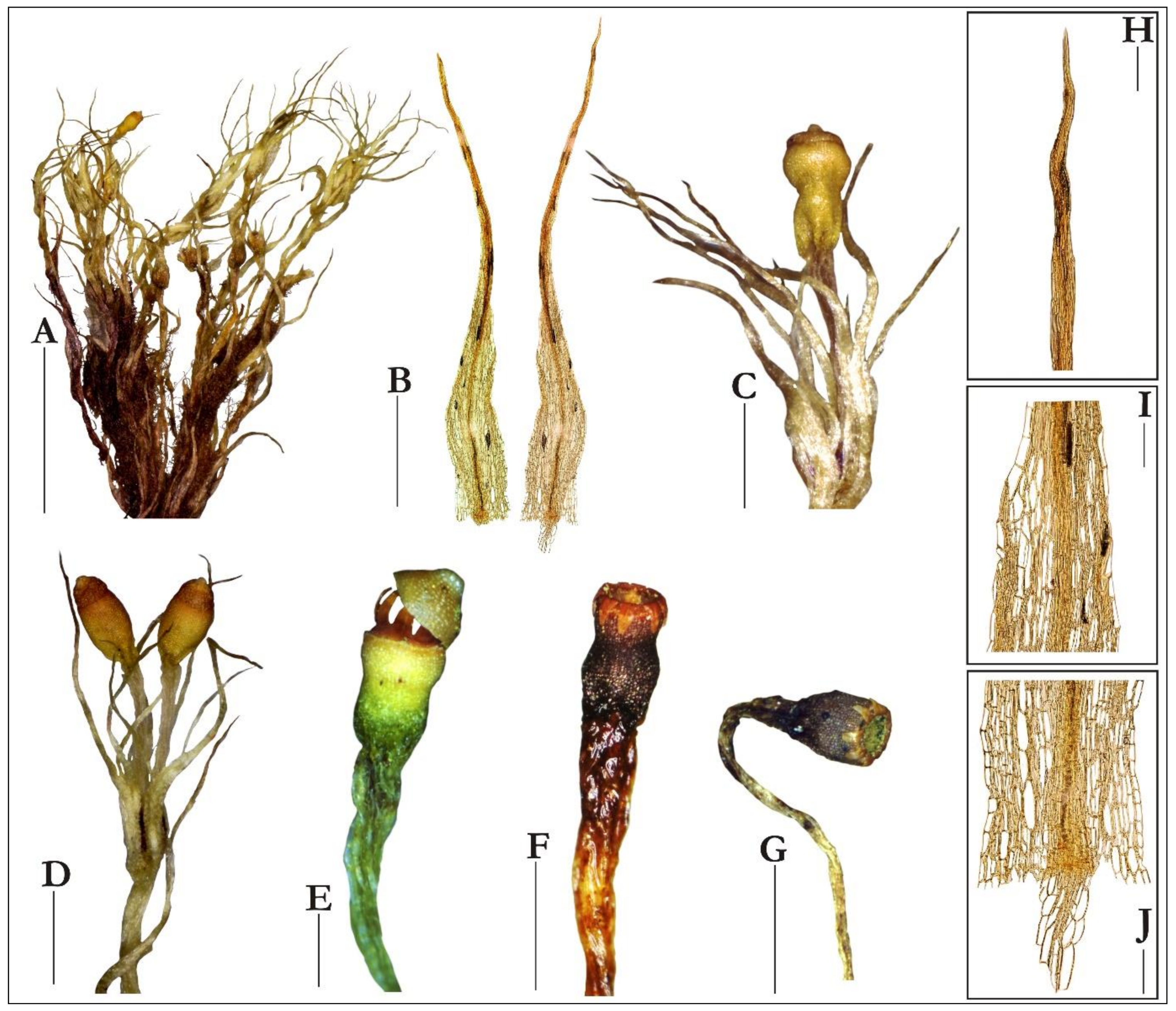The image is a detailed, abstract diagram showcasing various plant parts that are labeled from A through J. Each segment highlights different root structures and their distinct characteristics. Image A presents a bundle of wiry brown and white roots that are slightly bulbous at the ends. B depicts two more streamlined roots that curve gently upward. C displays a thicker root base with a bulb from which other roots branch out. D features two bulbs with roots spiraling around them, resembling bean sprouts. 

Image E shows a single, bulbous root that intriguingly looks like a Venus flytrap with spiky, tooth-like structures inside. F focuses on a darker, solitary bulbous root compared to the others. G consists of another spindly root with one bulb at the end. Lastly, H, I, and J illustrate the same root at different stages of growth, ranging from a super straight formation in H to increasingly chaotic, sprawling roots in J. The diagram is set against a white background, framed in black, and displays a rich variety of colors, including tan, gray, red, rust, and bright neon green. Despite its abstract nature, the diverse textures, shapes, and colors suggest a comprehensive study of varied root structures.